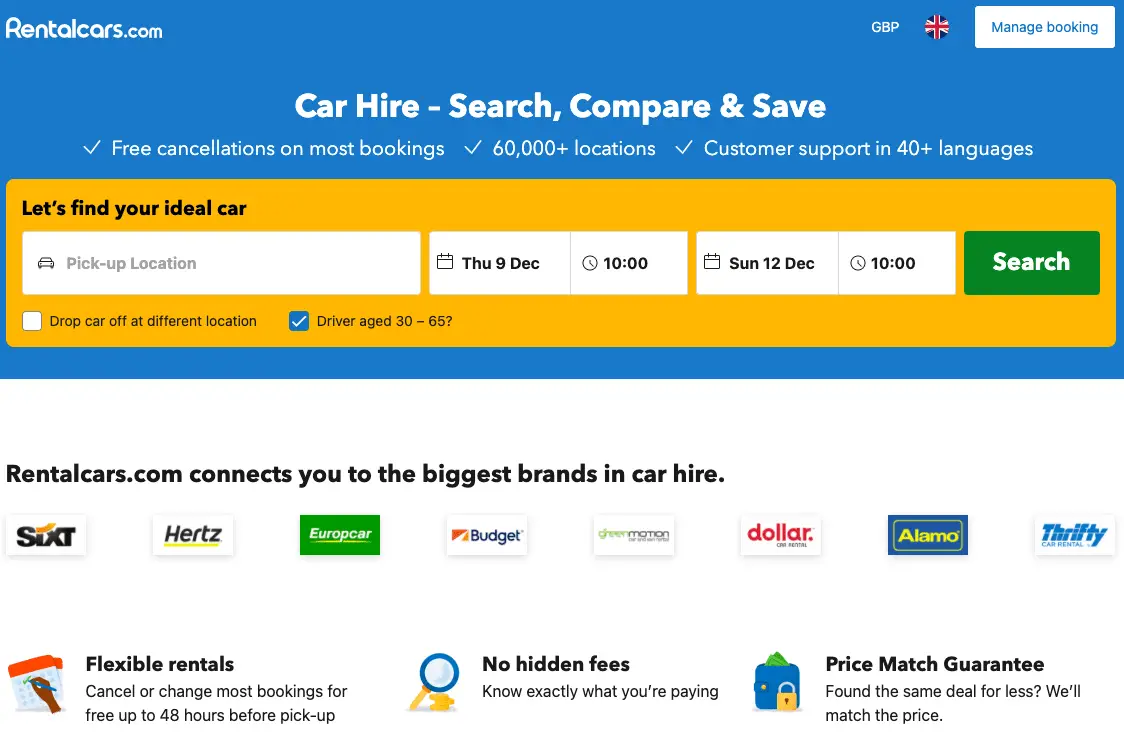The image depicts a promotional section from the rentalcars.com website. The background is predominantly blue. In the upper right corner, within a white box, are the words "Manage Booking," accompanied by a circular British flag icon and the abbreviation "GRP."

Central to the image is a prominent blue box with the text "Car Hire Search, Compare and Save." Below this, three key benefits are listed, each marked with a check mark: "Free Cancellations on Most Bookings," "60,000+ Locations," and "Customer Support in 40+ Languages."

Inside a gold bar, there are fields for entering the pickup location and dates, set from Thursday, December 9th at 10:00 AM to Sunday, December 12th at 10:00 AM. A green search button with white letters is placed at the end of this form. Options to check include "Drop off car at different location" and "Driver Age: 30 to 65," both marked as selected.

Below, a section highlights that rentalcars.com partners with major car rental brands including Sixt, Hertz, Europcar, Budget, Dollar, Alamo, and Thrifty. Further down, it emphasizes "Flexible Rentals" with the ability to cancel or change most bookings for free up to 48 hours before pickup, "No Hidden Fees" to know exactly what you’re paying, and a "Price Match Guarantee" to match any found deal for a lower price.